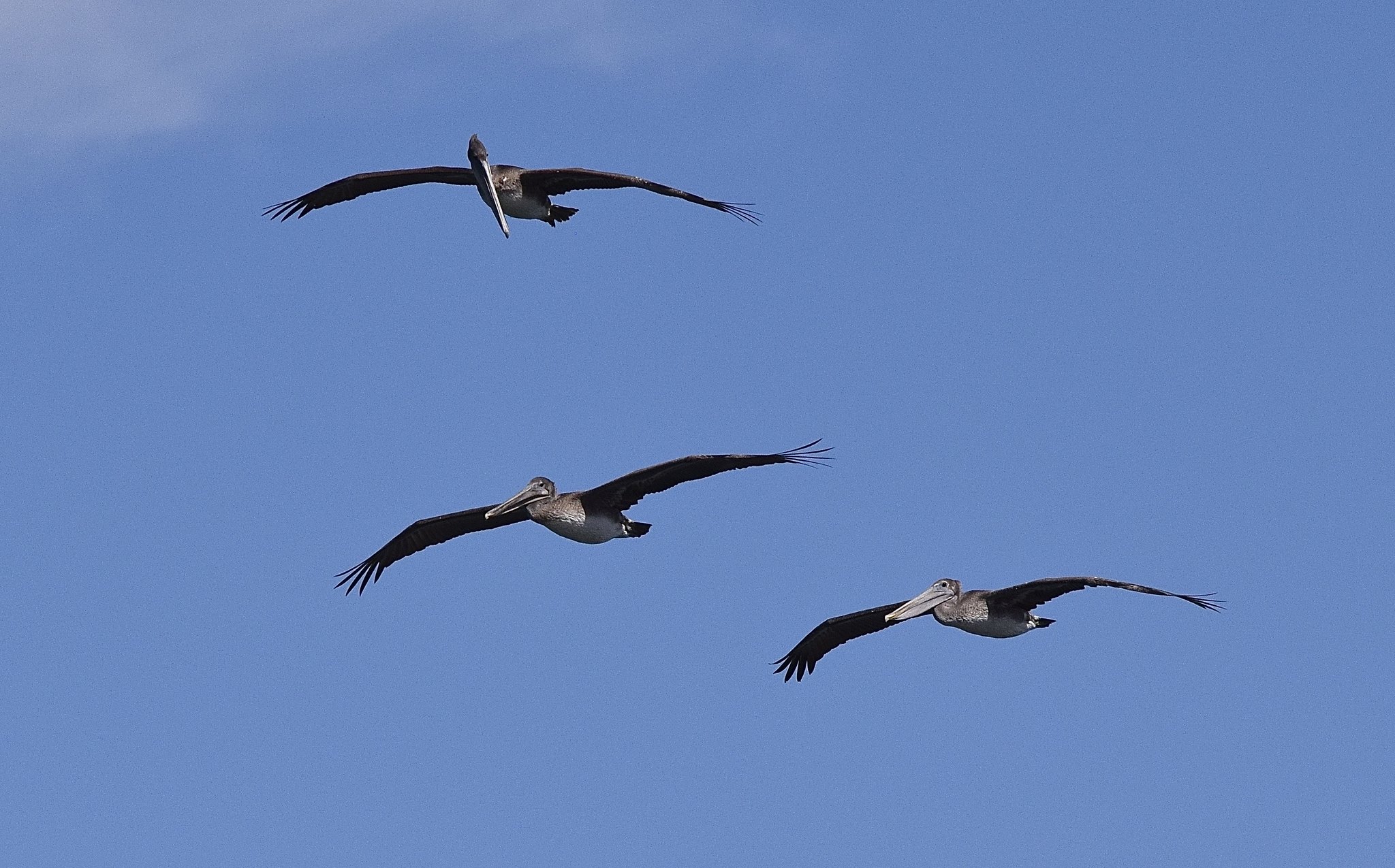In this image, we gaze up at a clear blue sky with hints of wispy, cirrus clouds scattering minimally across the expanse. The scene captures three large birds mid-flight, identified as pelican-like due to their distinctive features—a gray body, black wings with prominent wingtip feathers, and long, substantial beaks. The birds are soaring with their wings fully extended, creating an impression of grace and fluid motion. The topmost bird is casting its gaze downward at the two below it, which appear more focused on their direction of flight, with their eyes fixed to the left. Their legs are tucked beneath them, reducing air resistance. The composition showcases an open and expansive sky, emphasizing the freedom and space surrounding these magnificent creatures.